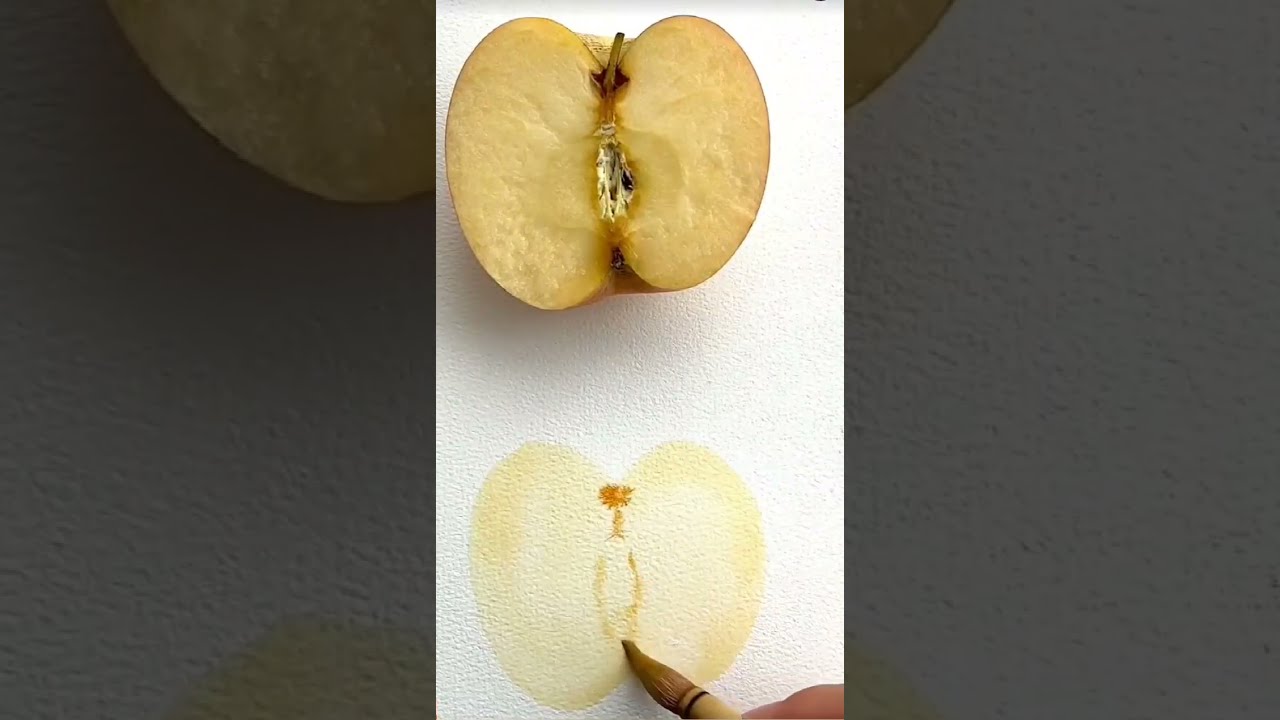In the center of the image, there is a prominent, cut-in-half apple resting on its rounded back on a piece of white striped paper. The apple displays a slightly oxidized cross-section, revealing its stem, seeds, and flesh. Directly below it, we see someone in the process of replicating the apple using a paintbrush. The artist has sketched the outline and started painting the inside of the apple, capturing the core and a bit of the stem. The background comprises a white striped section in the middle, flanked by darker, enlarged sections of the original photo of the apple, which are slightly darkened and provide a contrasting backdrop to the bright central composition. The right and left thirds of the image display portions of this enlarged and darkened apple image, giving the entire setup a layered, focused effect.